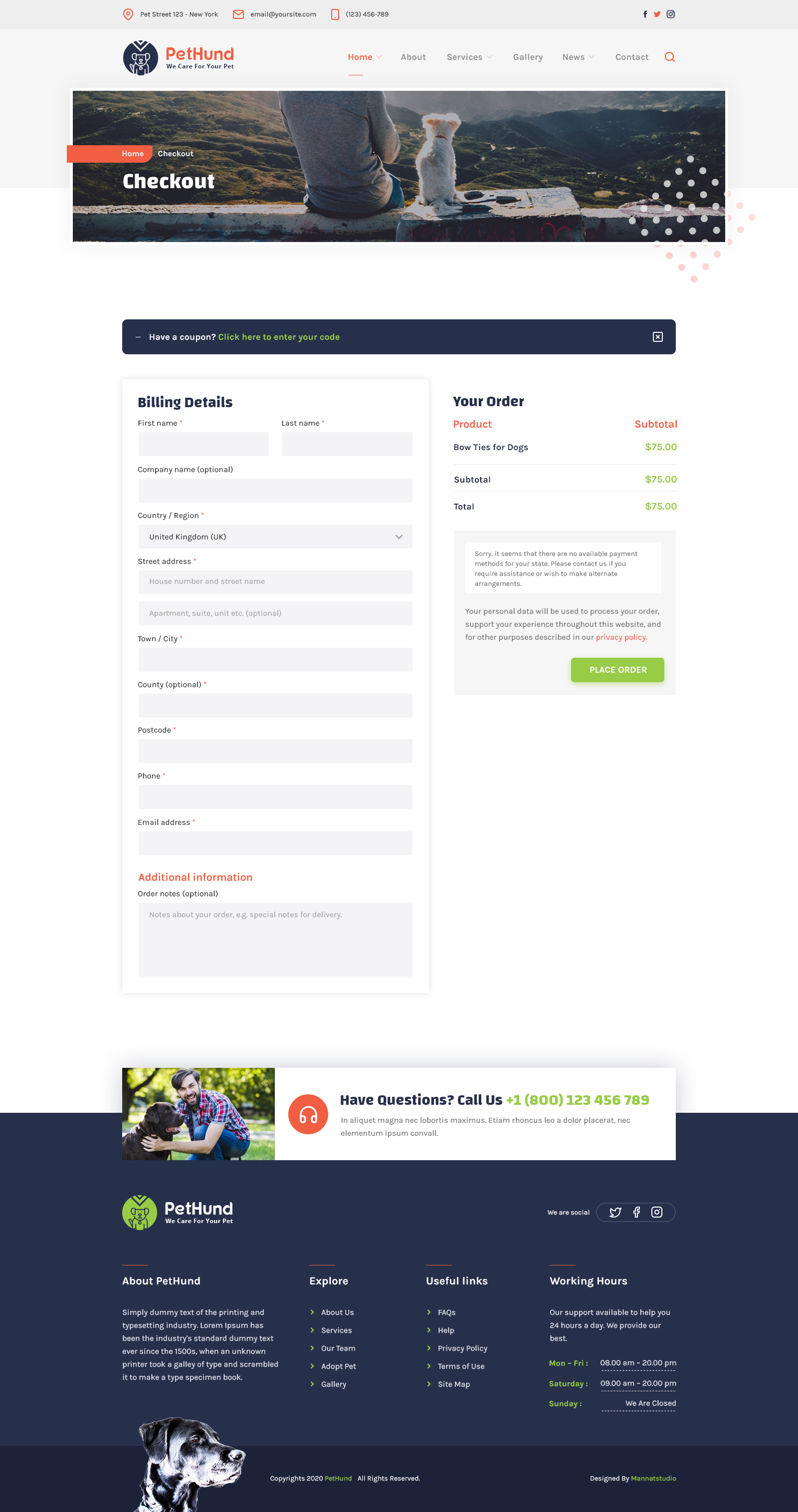The image captures a busy yet detailed webpage, likely a checkout page for an online pet supplies store named PetHud. 

In the upper left corner, the webpage has a grey background filled with indistinguishable text or design elements. On the upper right, recognizable social media icons for Facebook, Twitter, and Instagram are visible, hinting at the brand's online presence. "PetHud" is prominently displayed in bold, orangey text.

To the right, in grey text, there appears to be a hidden navigation link with the words starting with "Home," though the full text is too small to discern. Below, an image features a man in a grey shirt and blue jeans sitting on a stone wall. Next to him, a small white puppy gazes into the distance, both with their backs turned towards the camera, creating a serene and thoughtful moment.

On the left side of the page, the word "Checkout" is clearly written. Beneath this, the "Billing Details" section is highlighted in blue, featuring numerous grey boxes meant to be filled in with purchaser’s information. Though many details remain unreadable due to the small font size, pertinent labels indicate required details.

To the left, in a similar bluish color, the phrase "Your Order" can be seen at the top of a section that lists the order summary. Product names are listed on the left with their respective subtotals on the right. Despite the small print, one can discern repetitive items priced at $75 each.

At the bottom, a green button marked "Place Order" in white text urges completion of the purchase. The page concludes with additional text, likely contact information for PetHud, rendered in white at the very bottom.